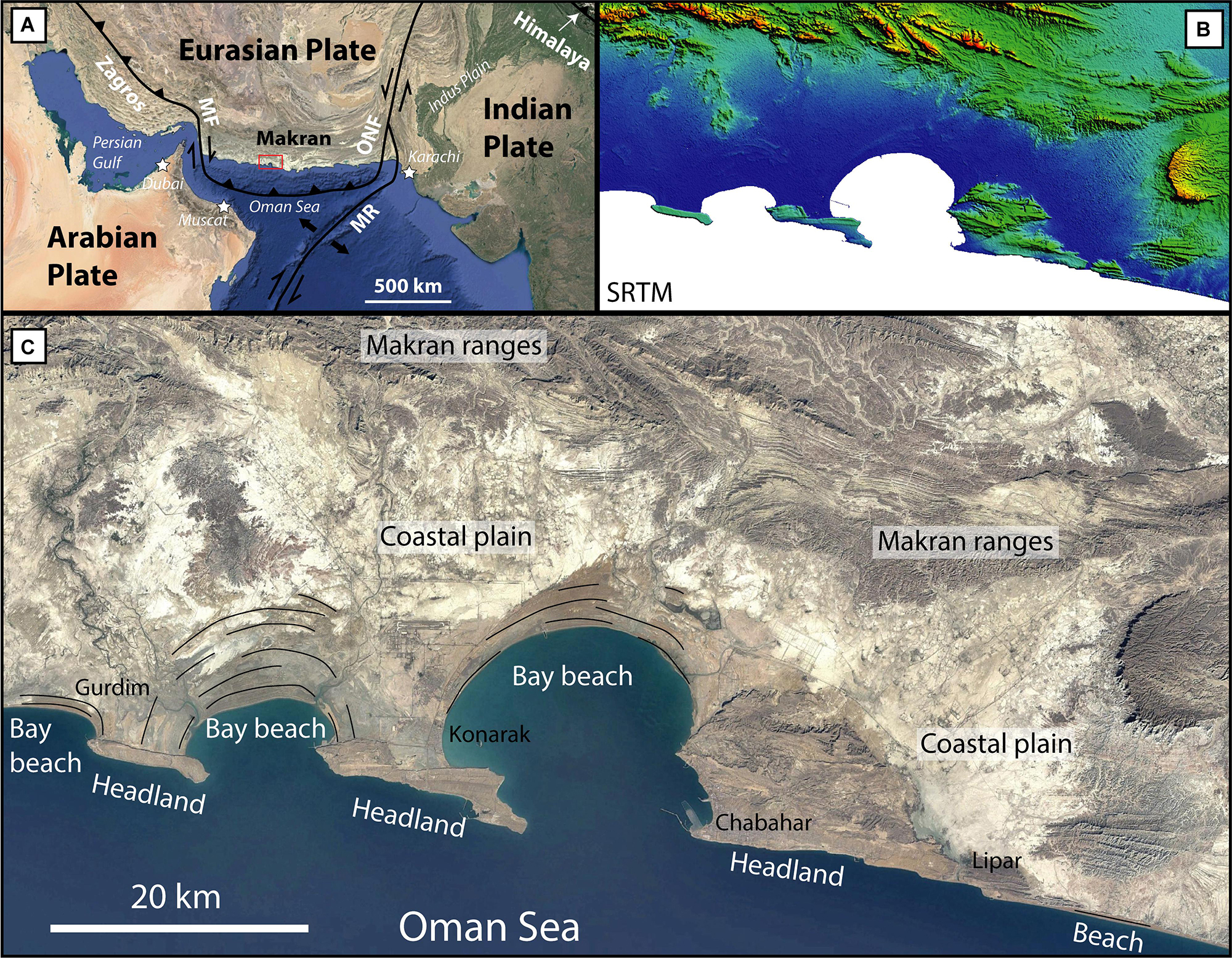The image features three detailed maps sectioned into three parts, with the largest map positioned at the bottom. The smaller, top-left map is labeled 'A' and depicts the Eurasian Plate, Arabian Plate, and Indian Plate, along with geographic features such as the Himalayas, Persian Gulf, and Oman Sea. The landscape appears varied, with brown areas indicating land and blue depicting water, and a scale of 500 kilometers is noted. The top-right map, labeled 'B,' presents a different type of map with a notable amount of green, suggesting significant rainfall or vegetation, but lacks specific labels except for "SRTM." The large bottom map, labeled 'C,' encompasses the vast region of the Eurasian Plate north of the Oman Sea, highlighting the Makran Ranges, Coastal Plain, Bay Beach, and numerous mountain ranges and plains, using a closer scale of 20 kilometers. The maps are graphically enclosed within white boxes outlined in black, providing a comprehensive visualization of the geographic and topographic details of the regions depicted.